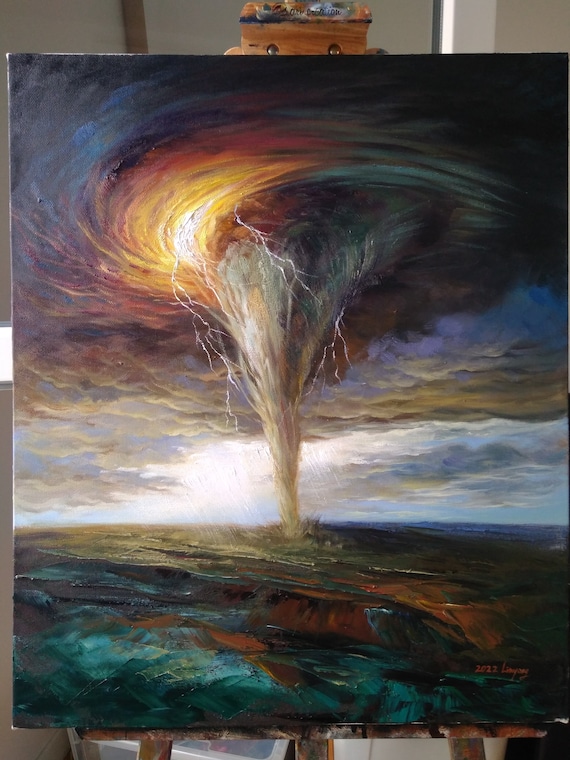The photograph captures a large, vibrant painting mounted on a wooden easel, which is partially visible beneath the canvas. The scene depicts a dynamic tornado, characterized by a thin funnel at the bottom and a expansive, swirling cloud formation at the top. Lightning streaks from the yellow and orange segments of the cloud into the twister below. The painting's backdrop features a vividly detailed sky with scattered clouds and bright sunlight, transitioning into a cyan blue landscape marked by rust and orange hues. The tornado appears to be forming over a large body of water, distinguished by dark grayish-blue tones accented with dark orange highlights. The bottom right corner of the painting is signed "2022" followed by an unclear name beginning with an 'L'. The entire artwork exudes a sense of movement and intensity, rendered with a palette of bright, contrasting colors. In the background, beneath the easel, white storage totes with clear lids are visible, hinting at the artist’s organized workspace.